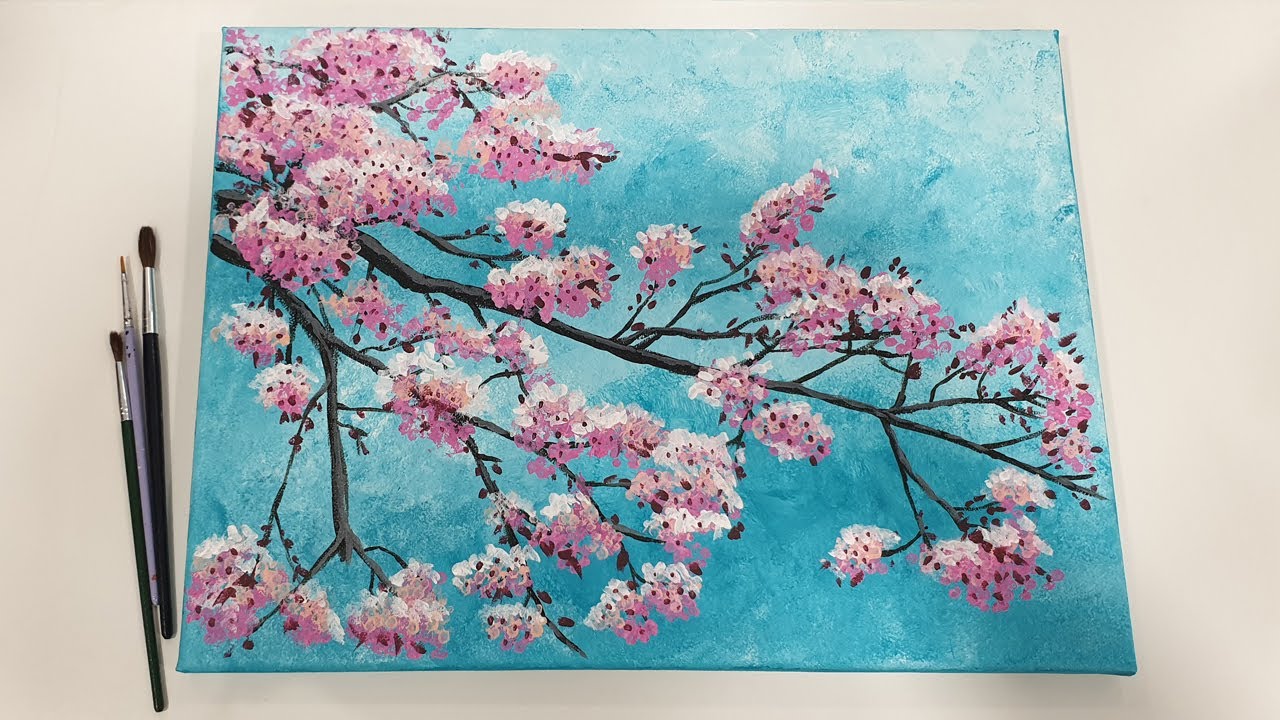The photograph captures a detailed watercolor painting resting on a large white table. The painting prominently features a large limb of a cherry tree extending from the left side towards the right, with numerous branches adorned with clusters of pink, white, and red cherry blossoms in full bloom. The flowers are depicted in varying sizes, creating a lush and textured portrayal of springtime. The background is a rich blue sky, rendered with a textured finish and subtle cloud patterns, enhancing the natural beauty of the scene. To the left of the painting, there are three paintbrushes: two with black handles and one with a blue handle, all lying parallel to each other. The paintbrushes have black handles with silver ferrules holding the bristles. This painting beautifully captures the essence of spring with its vibrant blossoms and serene blue sky.